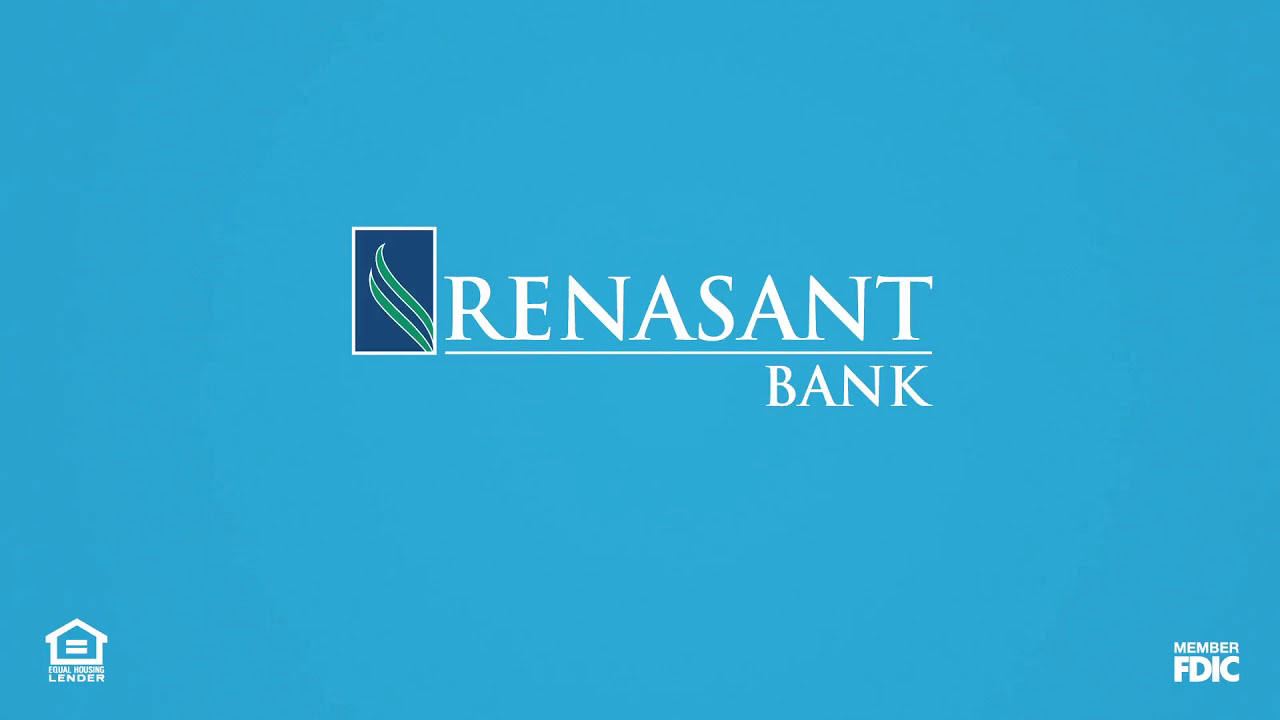This image features a predominantly blue background, with prominent white text and symbols. At the center of the image, large, all-capital letters spell out "RENAISSANCE BANK," with "RENAISSANCE" slightly larger than "BANK" and an underline beneath "RENAISSANCE." To the left of "RENAISSANCE," there is a navy blue, vertical rectangle outlined in white, containing the bank's logo: two green diagonal lines resembling grass blades or vines. At the bottom left corner, an icon of a house with an equal sign underneath it indicates "Equal Housing Lender" in white text. Similarly, in the bottom right corner, also in white text, are the words "Member FDIC." This image appears to be an advertisement or a section from a website providing information about the bank.